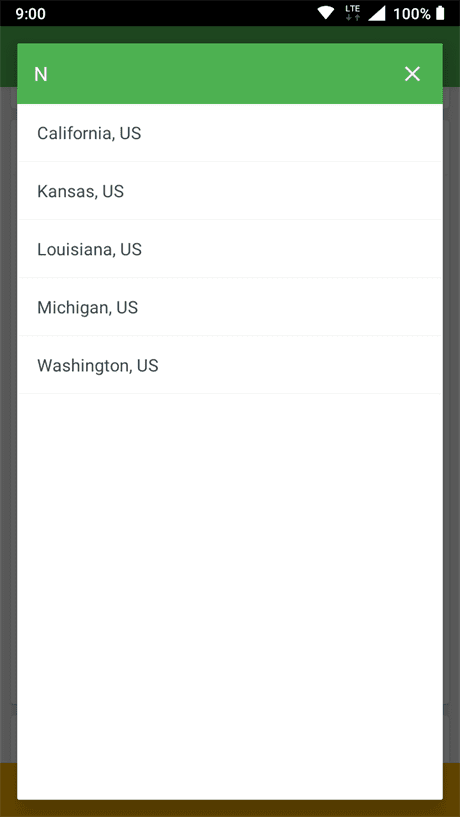This image is a detailed screenshot of a pop-up page displayed on a mobile phone. The backdrop behind the pop-up is quite blurred and enveloped in darkness, contributing to a dim overall appearance. 

At the top of the phone's interface is a black notification bar featuring white text and icons. On the left side, the current time is displayed as "9:00". The top right corner houses five icons: a white Wi-Fi symbol, the text "LTE" accompanied by two gray arrows (one pointing down, the other up), a white triangle icon, the battery percentage indicated as "100%", and a fully white battery icon. 

Beneath this notification bar is the pop-up window. The pop-up features a white backdrop and a green header. To the left of the green header, a white "N" is visible, and to the far right, a white "X" marks the close option. The white background of the pop-up contains listed locations separated by thin, light gray lines. The locations are presented in dark gray text and listed as follows:
- California, U.S.
- Kansas, U.S.
- Louisiana, U.S.
- Michigan, U.S.
- Washington, U.S.

A final thin gray line differentiates these locations from the remaining portion of the pop-up, which is just an expanse of pure white negative space, devoid of any content or elements. 

In the dim background, part of the underlying webpage is faintly visible. The page consists of a gray body, a header in a similar shade of green (darkened due to the overall darkness of the image), and an orange footer at the bottom.